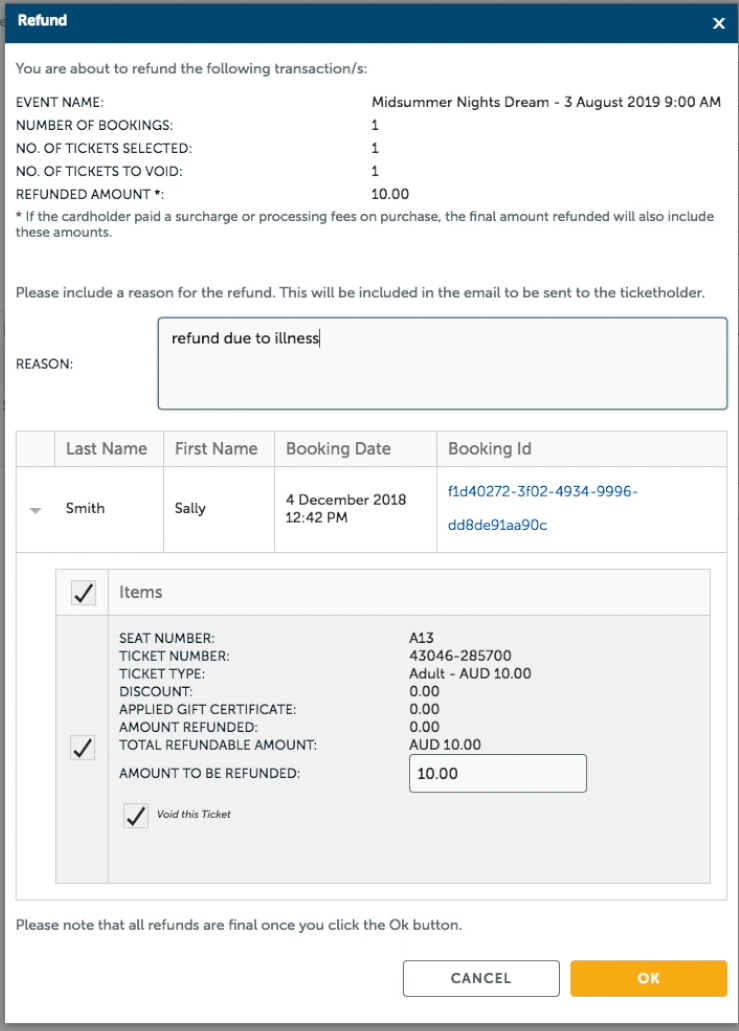Screenshot of a Refund Page for Tickets:

The image displays a detailed screenshot of a refund confirmation page for a ticketing system. The page features a clean design with a predominantly white background and a blue banner at the top that prominently reads "Refund."

Below the banner, the text informs the user that they are about to refund the following transactions:
- **Event Name:** Midsummer Night's Dream
- **Date:** 3 August 2019, 9 a.m.
- **Number of Bookings:** 1
- **Number of Tickets Selected:** 1
- **Number of Tickets Voided:** 1
- **Refunded Amount:** $10

Additionally, the page clarifies that if the cardholder paid any surcharge or processing fees at the time of purchase, these amounts will also be included in the total refund.

There is a section that allows the user to enter a reason for the refund, which will be sent via email to the ticket holder. In this case, the reason provided is "Refund due to illness."

The user details are:
- **Last Name:** Smith
- **First Name:** Sally
- **Booking Date:** December 4th, 2018 at 12:42 p.m.
- **Booking ID:** Highlighted in blue, but the actual ID number is not visible in the screenshot.

The "Items" section includes specific information about the ticket:
- **Seat Number** (not specified in the description)
- **Ticket Number** (not specified in the description)
- **Ticket Type** (not specified in the description)
- **Discount Applied** (if any, not specified in the description)
- **Gift Certificate** (if any, not specified in the description)
- **Amount Refunded**: $10
- **Total Refundable Amount**: $10
- **Amount to be Refunded**: $10

There is a checkbox option to void the ticket, which is selected. A note at the very bottom of the page states, "Please note that all refunds are final once you click the OK button." 

The footer contains two action buttons: "Cancel" and "OK," with the "OK" button highlighted in orange.